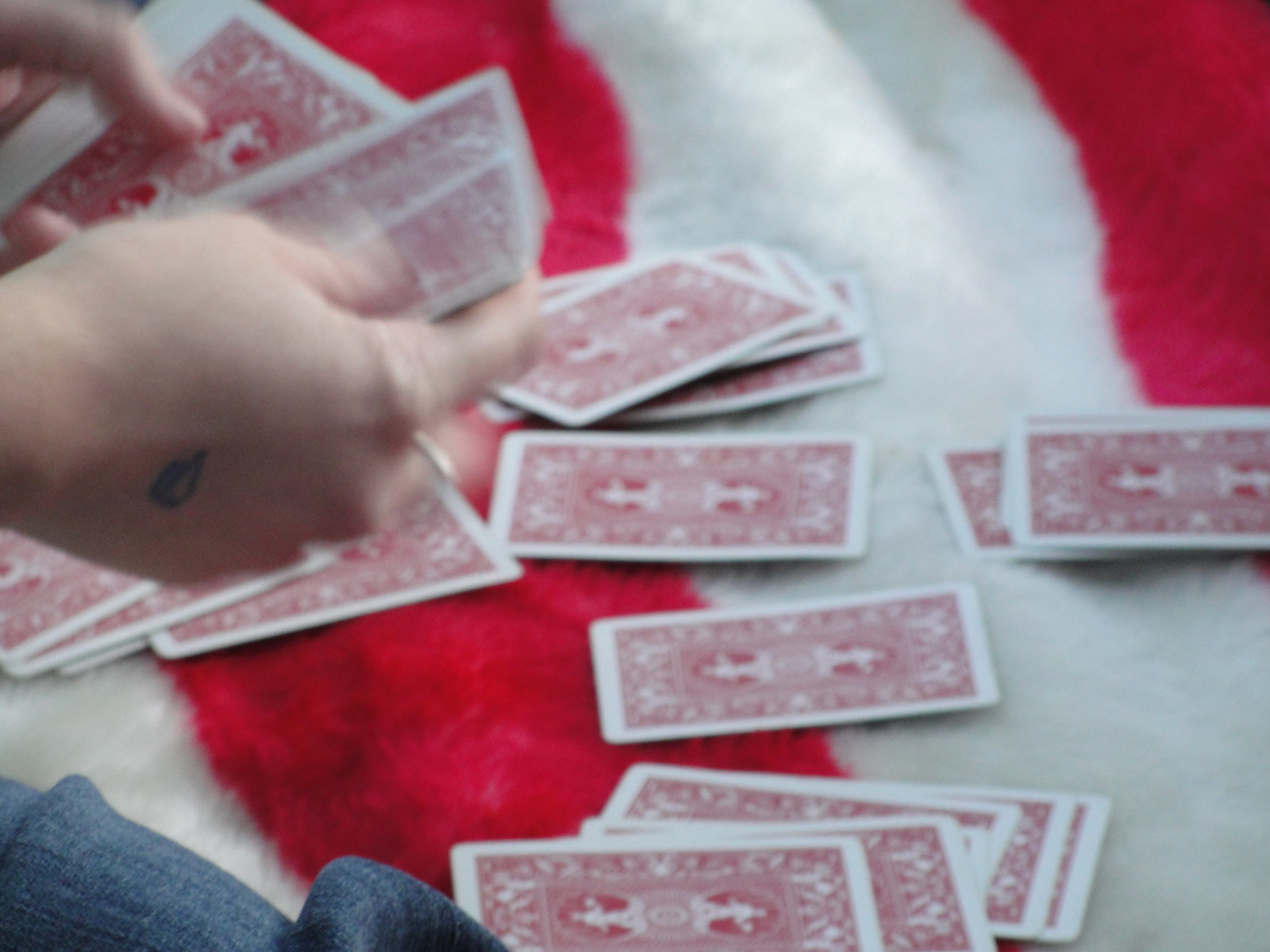The photograph is a blurred image depicting a Caucasian individual, whose gender is indeterminate, engaged in sorting playing cards. The background appears to be a red and white fluffy duvet or tablecloth. The person's left hand, adorned with a small teardrop tattoo near the knuckles, emerges from the top left of the frame, holding a packet of playing cards with a white border and intricate red design. The right hand is in the process of extracting a card from the pack and placing it onto one of several organized piles on the surface. The arrangement of these piles suggests a deliberate method of allocation. Additionally, a piece of denim fabric is visible in the bottom left corner, possibly belonging to the individual handling the cards.